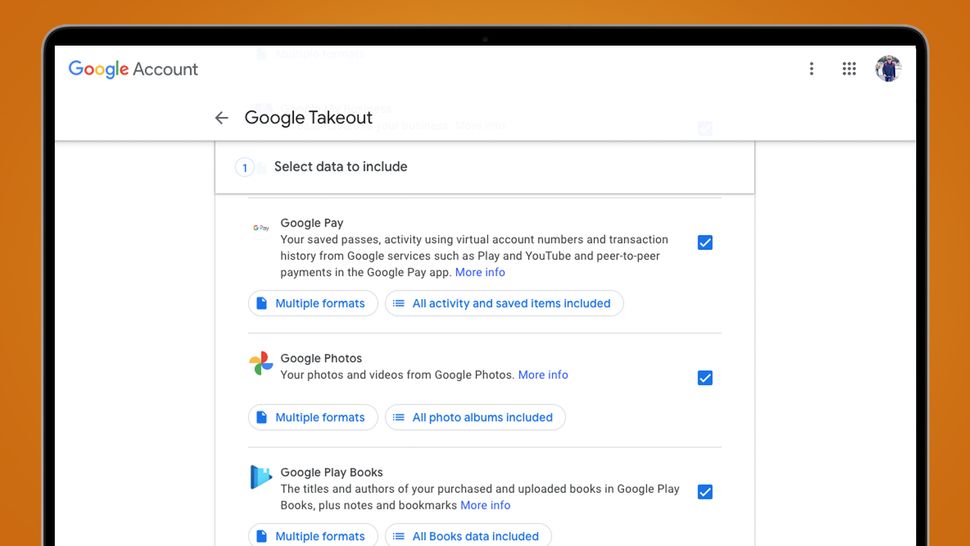The image captures a Google Account page displayed on a tablet, possibly a Samsung device, identifiable by the visible brownish-orange borders. The device's screen shows the Google Account interface prominently titled "Google Account" at the top-left corner. In line with modern design, the right-hand side features three dots (likely a menu icon), a grid of nine squares (possibly an app launcher), and a profile image depicting an indiscernible person.

On the left side, about mid-screen, an arrow icon points left, suggesting navigation options. A heading reads "Google Takeout," accompanied by a brief divider. Below it, a circled number "1" in blue indicates the first step, "Select data to include." Further down the screen, another section titled "Google Pay" explains the usage of virtual account numbers and transaction history from Google services like Play, YouTube, and peer-to-peer payments, with a "More info" link.

Following this, the image shows further sections for "Google Photos" and "Google Play Buttons." Each of these sections includes interactive elements corresponding to "multiple formats" and "all photo albums" options, indicating comprehensive data management features.

The background of the image is only partially visible due to the tablet's partial visibility, emphasizing the screen content.